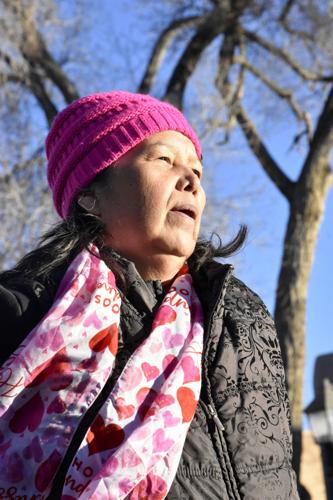The photograph features a middle-aged woman with light brown skin, possibly of Native American or Asian descent, seen from a right-side view. She is wearing a pink beanie and a matching pink, red, and white scarf adorned with hearts. Her long black hair cascades down past her shoulders and she has a silver earring in her right ear. Draped in a dark gray jacket with subtle floral designs, the woman stands against a backdrop of a clear blue sky and a large, mostly leafless tree, suggesting the photo was taken in late fall or winter. The sunlight illuminates her as she looks upward to the top right with a neutral expression. The overall composition maintains a photographic realism.